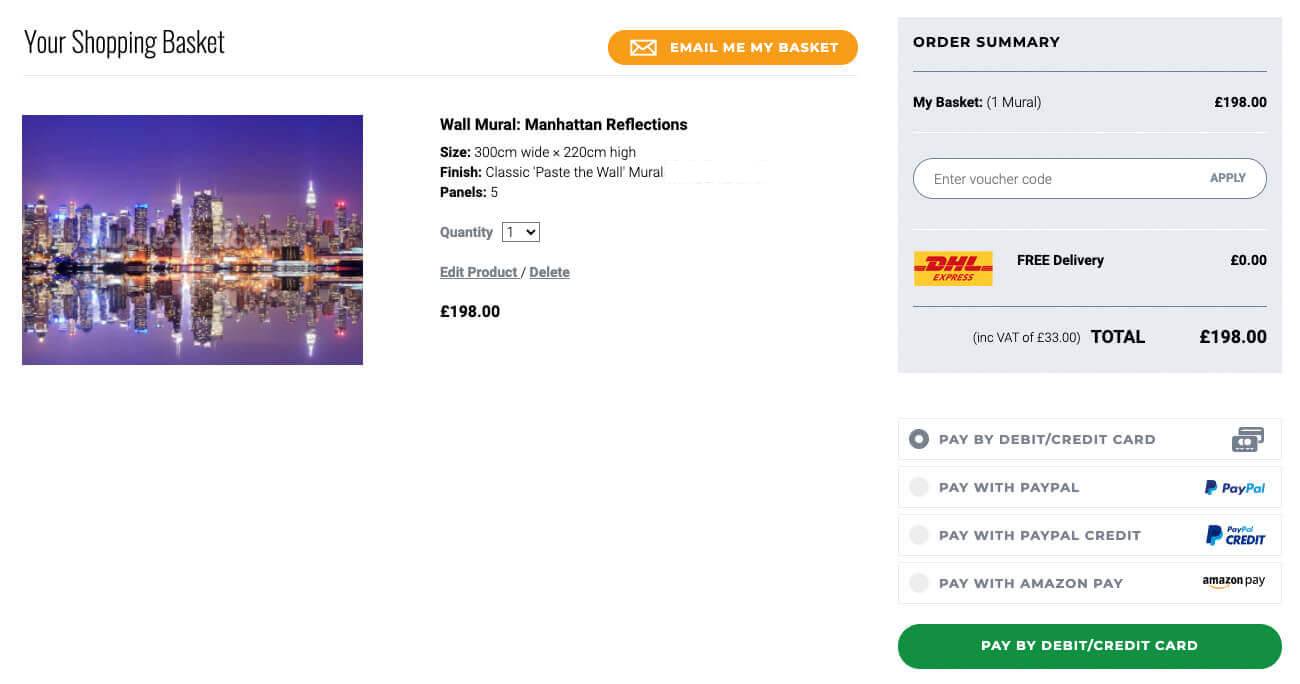This detailed caption corresponds to the image described:

"A screenshot of an online shopping basket displays the user's current order. At the top left, the page header reads 'Your Shopping Basket', accompanied by an orange banner with white text that says 'Email me my basket'. The main item in the basket is a wall mural titled 'Manhattan Reflections', featuring a purple-hued image of the Manhattan skyline reflected in water, illuminated by city lights. The mural measures 300 centimeters wide by 220 centimeters high, with a finish described as 'classic paste the wall mural panels'. The quantity of the mural ordered is one, and there are options to edit or delete the product. The mural costs $198.00.

To the right, an 'Order Summary' box outlines the order details, listing 'My Basket: 1 Mural - $198.00'. There is a field available for entering a voucher code. The delivery service is DHL Express, indicated by a red and yellow box, which offers free delivery. The total order cost is $198.00.

Below the order summary, there are four payment options: 'Pay with Debit/Credit Card', 'Pay with PayPal', 'Pay with PayPal Credit', and 'Pay with Amazon Pay'. A green banner at the bottom of the screen highlights the selected payment method, which is 'Pay by Debit/Credit Card'."